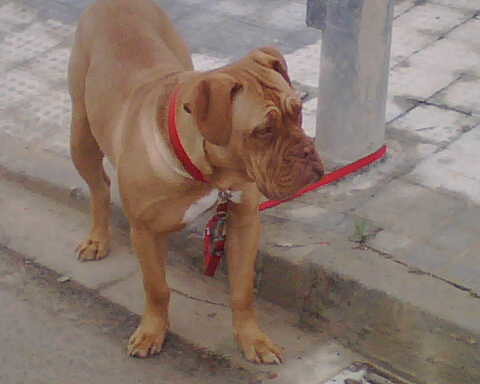The image depicts a light brown pit bull, possibly mixed with Mastiff, standing on a sidewalk tied to a pole with a red leash and collar. The scene is set on a street with a sidewalk comprised of pale-colored, square tiles, some of which appear slightly wet, suggesting it might have rained recently. The dog stands on all four paws and gazes off to the right side of the image. In the lower right corner, the edge of a drain can be seen. The sidewalk elevates slightly from the street on the left, creating a clear separation between the two surfaces.